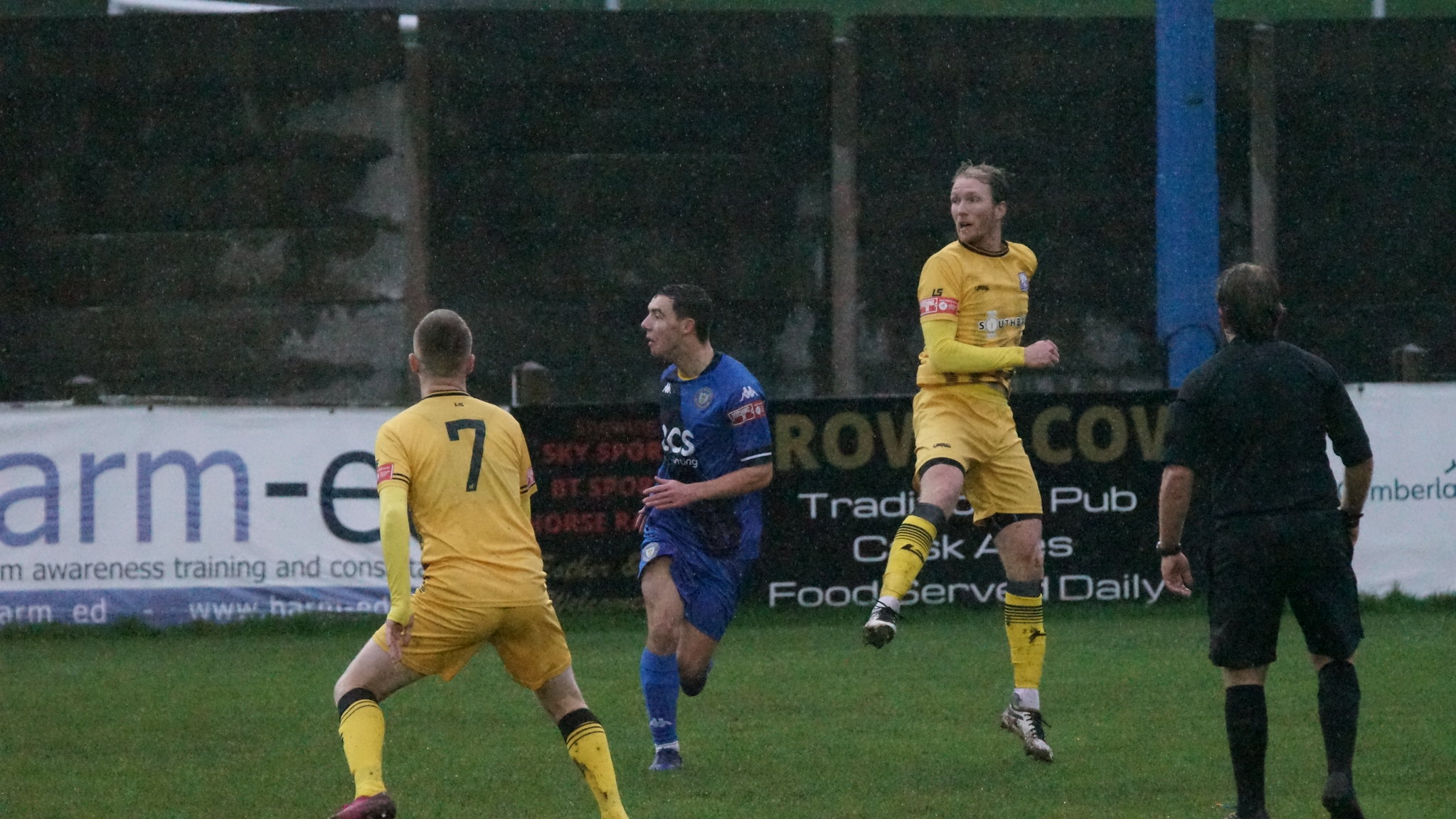This photograph captures an intense moment at a soccer game. From left to right, we see a player in a yellow jersey with the number seven on his back, poised to run, his legs spread wide. To his right is a player in a full blue uniform—shirt, shorts, socks, and shin guards—caught mid-run, looking to the left. Next to him is another player in yellow, caught in mid-air with one leg lifted and the other toe barely touching the ground, as if he's jumping. On the far right, a referee dressed in black—shirt, shorts, and socks—looks on, also facing away from the camera. All players are intensely focused on something to the left, possibly the ball not in frame. They stand on a green field, which could be grass or turf. Behind them, a large concrete wall adorned with various advertising posters forms the background. Despite partial obstructions, one poster reads "Arm E Awareness Training" with white, blue, and black lettering, while another mentions a trading pub with food service, in white and gold lettering on a black background. The quality of the image suggests either poor lighting or raindrops, adding to the dynamic atmosphere of the scene.